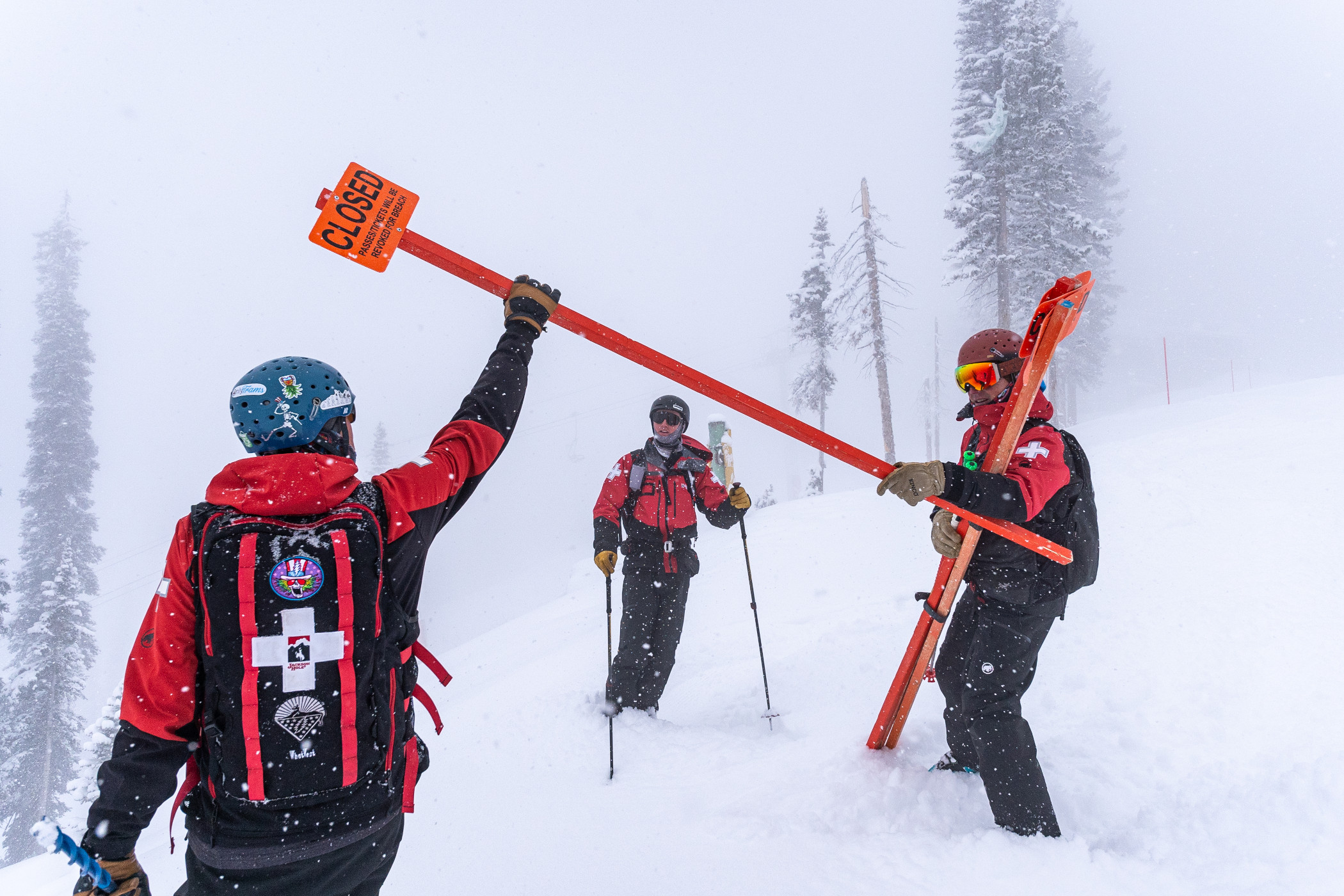In this snowy, daytime scene taken at a ski resort, three men outfitted in matching red and black snow gear are hard at work amidst a near-whiteout. They wear safety helmets and ski goggles, with their red jackets featuring a distinctive white first aid cross on the sleeves and their black pants offering further contrast. Each man carries a black backpack adorned with red stripes and a white cross, adding to their uniform look as ski patrol members. 

The central figure holds a long orange pole bearing an orange "CLOSED" sign with additional text warning that passes and tickets will be revoked for breaches. His position near the top of the hill, which slopes from the top right to the bottom left, hints at their activity of marking restricted ski areas. One man stands to the right, holding a similar sign, while the man in the center, stationed between his colleagues, steadies himself with ski poles despite no skis being visible. Their surroundings are blanketed in thick snow, obscuring visibility and offering only glimpses of a few pine trees in the background. Despite the challenging conditions, the ski patrol team appears focused on ensuring the safety of the resort's visitors.